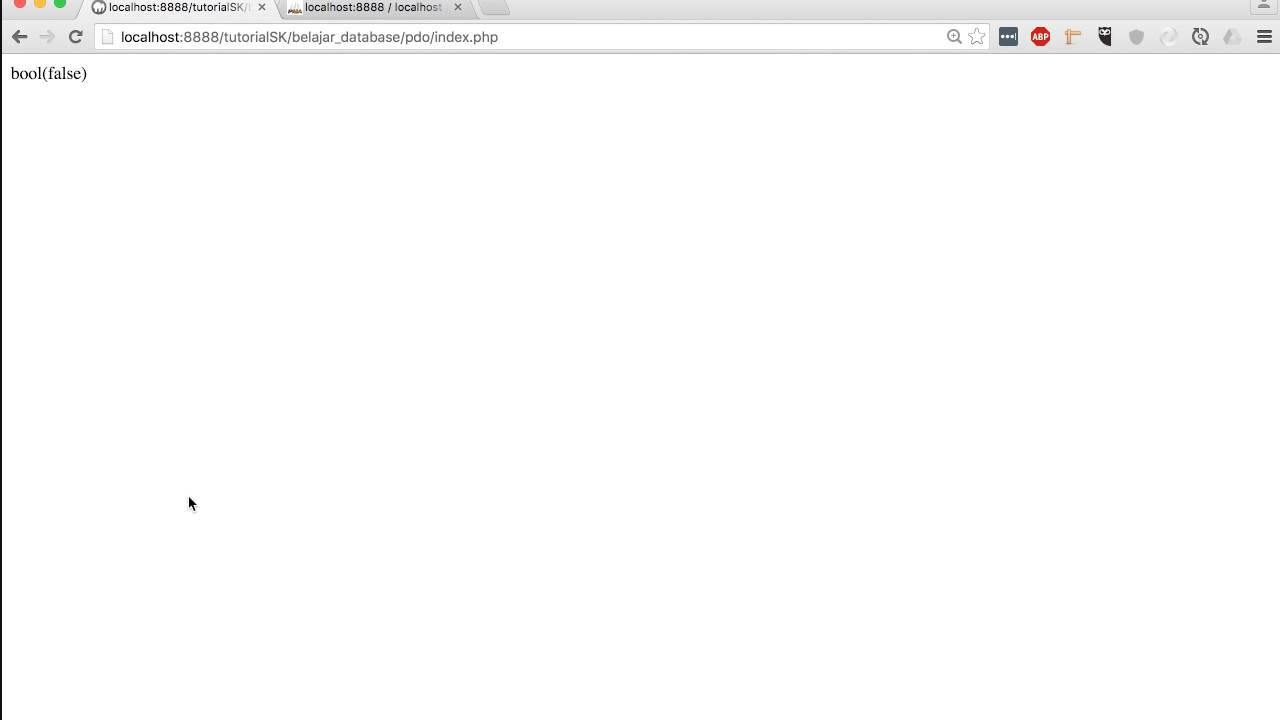The image is a horizontally rectangular screenshot of a computer monitor, capturing the browser window with two tabs open at the top. The active tab is titled "localhost:8888/tutorialSK," with a portion of the title obscured. The second tab reads "localhost:8888/localhost." Below the tabs, the browser's navigation bar displays the back, forward, and refresh icons on the left. The URL in the address bar is "localhost:8888/tutorialsk/belajar_database/pbo/index.php."

The main content area of the screenshot is mostly blank, except for a small detail in the upper left section, which displays "bool (false)" in parentheses. Additionally, in the bottom left quadrant of the image, the mouse cursor is visible, pointing upward towards the upper left corner of the screen.

This detailed caption provides a comprehensive description of the visual elements present in the screenshot.